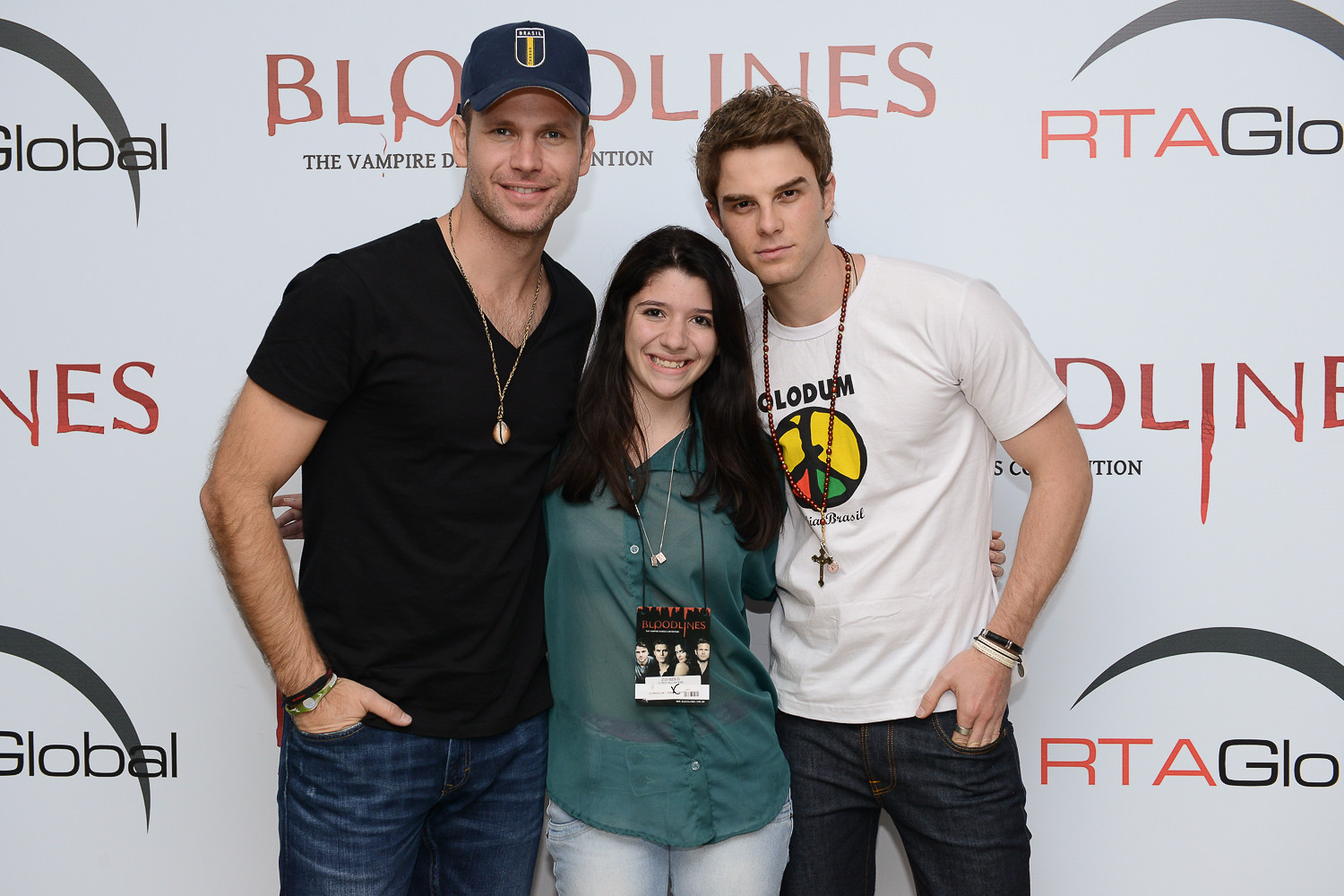The image captures three individuals posed in front of a promotional backdrop, likely at a red carpet event for a TV show or movie. The backdrop prominently displays "Bloodlines" and "RTA Global" written across it. The group consists of two men and a woman. The man on the left is dressed in a short sleeve black shirt, blue jeans, a long necklace, and a blue baseball cap. The woman in the middle, who has long dark brown hair and appears shorter than the men, is wearing a sheer green top, light blue jeans, and two necklaces—one with a small pendant and the other displaying a card linked to the "Bloodlines" movie. The man on the right sports a short sleeve white shirt adorned with a peace sign, blue jeans, and a very long cross necklace. Both men have their hands in their pockets, while the woman has her hands around her neck. All three individuals have light skin tones, and they are all smiling for the camera, except for the man on the right who has a more solemn expression.